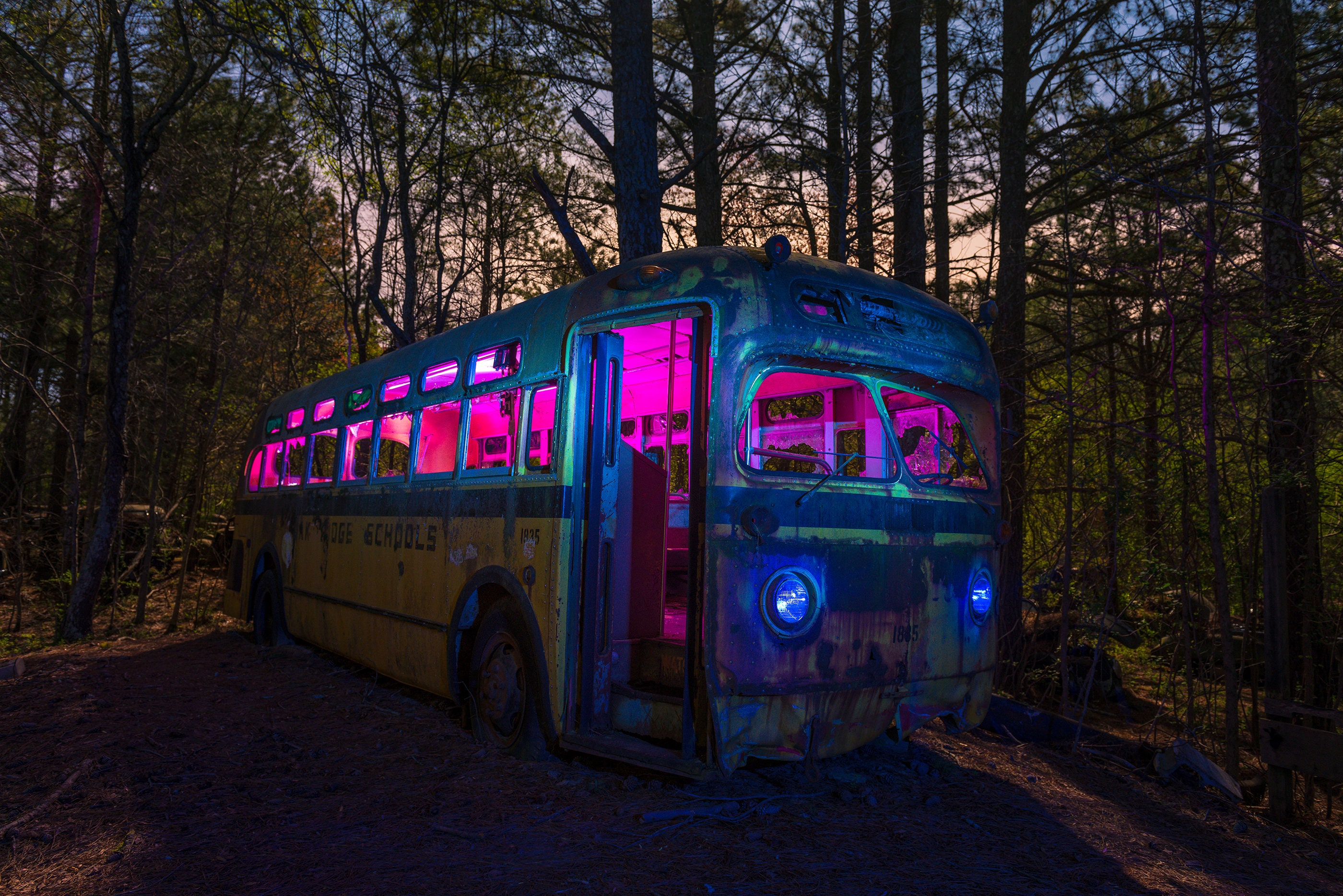The photograph showcases an abandoned and dilapidated school bus that appears to be positioned diagonally in the center of a forest scene. The bus, facing towards the bottom right, exhibits a weathered exterior with its yellow paint at the bottom and a grey-streaked upper section, likely due to years of exposure and neglect. The surface of the bus is coated in a thick layer of dust, hinting at its long-term abandonment.

The bus seems to possess a haunting yet intriguing ambiance, partly because of the unusual pink neon light emanating from its interior, casting a surreal glow through the windows. Complementing the eerie pink glow are two blue, rounded headlights at the front. The ground underneath and around the bus appears elevated, covered in a mix of grey and brown dirt, which adds to the rustic and abandoned feeling of the scene.

Surrounding the bus are tall trees, their dense foliage framing the vehicle and enhancing the sense of isolation. Above the trees, glimpses of the sky show a blend of blue and cream hues, suggesting the time might be either early morning or late evening, as indicated by the subtle, diffused lighting. The combination of the abandoned bus in disrepair with the surrounding woodland creates a striking and somewhat mysterious visual narrative.